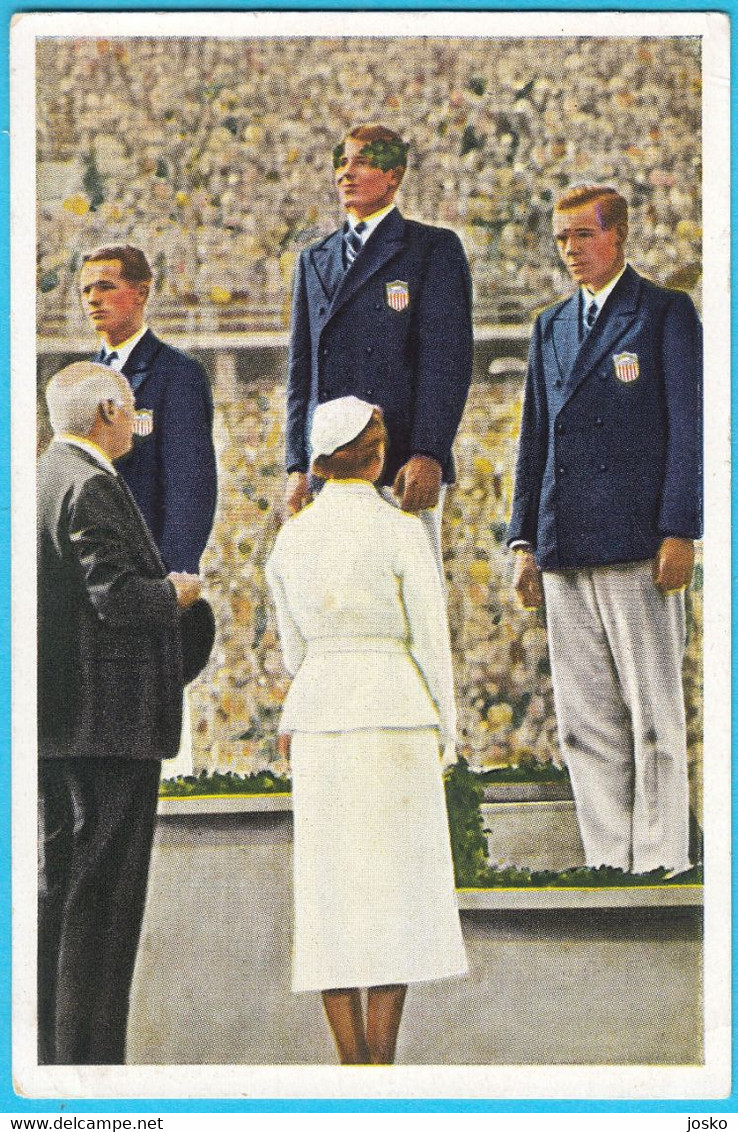This color image, possibly from the 1930s or 1940s and resembling a photograph or a painting found in a newspaper ad, captures an Olympic medal presentation set against the backdrop of a vibrant arena filled with spectators. Centered on a tiered podium resembling a first, second, and third place arrangement, three young Caucasian men stand proudly. The middle athlete, elevated higher than the others, wears a blue jacket adorned with a red, white, and blue patch on the left pocket, white pants, a white shirt, a blue and white striped tie, and a laurel wreath on his head, indicative of Olympic victory. Flanking him are two other medalists dressed similarly. 

In the foreground, a man in a black suit, carrying a hat, stands beside a woman adorned in an all-white outfit complete with matching white skirt and hat. She has brown hair and faces the athletes with her back to the camera, as if poised to present medals. The image also features text at the bottom reading "www.dellcampi.net" and to the right, "JOSCO."